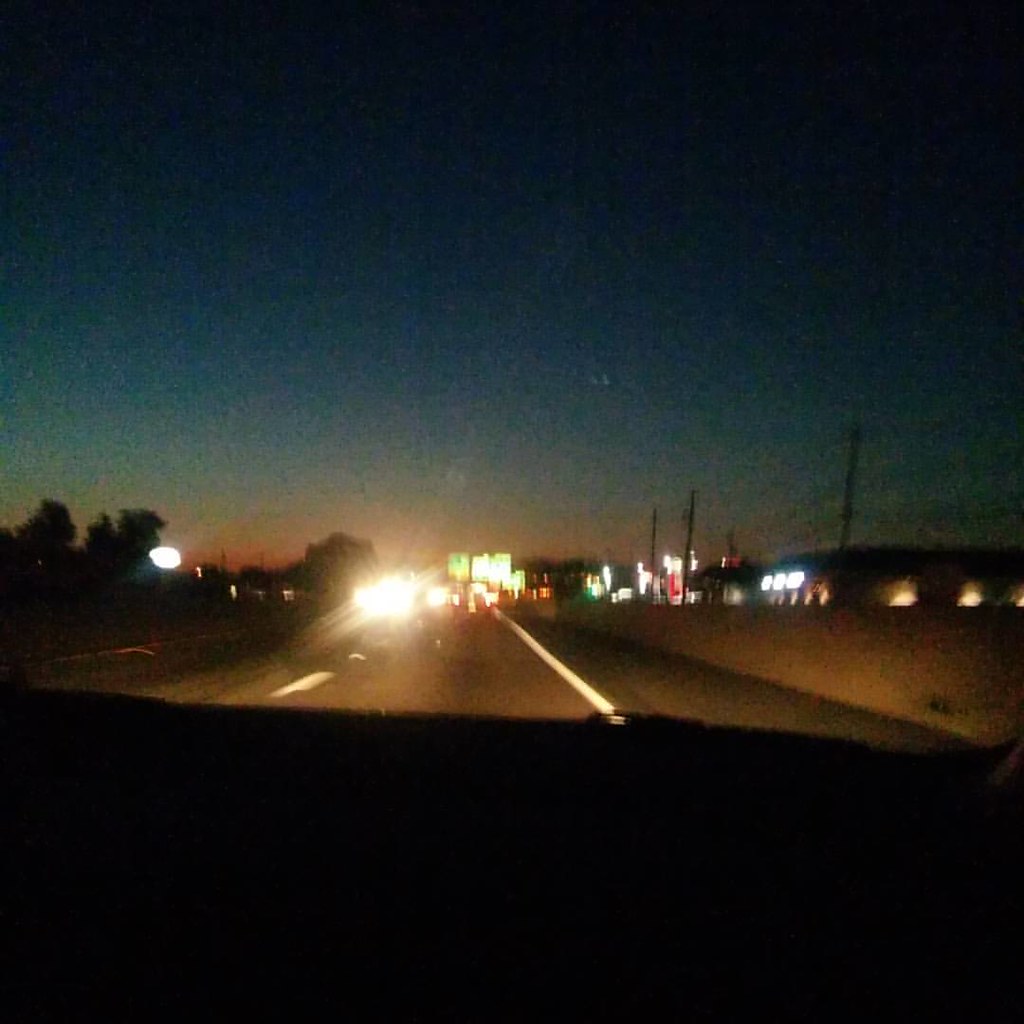A blurry nighttime scene captured from the viewpoint of a car's windshield, as it traverses a two-lane road. The white centerline and dashed stripes of the road stretch out into the distance, guiding the way. Oncoming cars with bright, slightly distorted headlights approach, adding a sense of movement and urgency to the scene. To the right, the road shoulder extends into the darkness, punctuated by scattered telephone poles that march off into the distance. The right side is illuminated by the occasional lights from businesses closer to the roadside and more distant ones fading into the horizon. Overhead, the dimly lit sky transitions from a faint glow at the horizon to a deep, encompassing darkness as it rises. The image captures an atmosphere of late-night travel, marked by the interplay of artificial lights and the encroaching night.